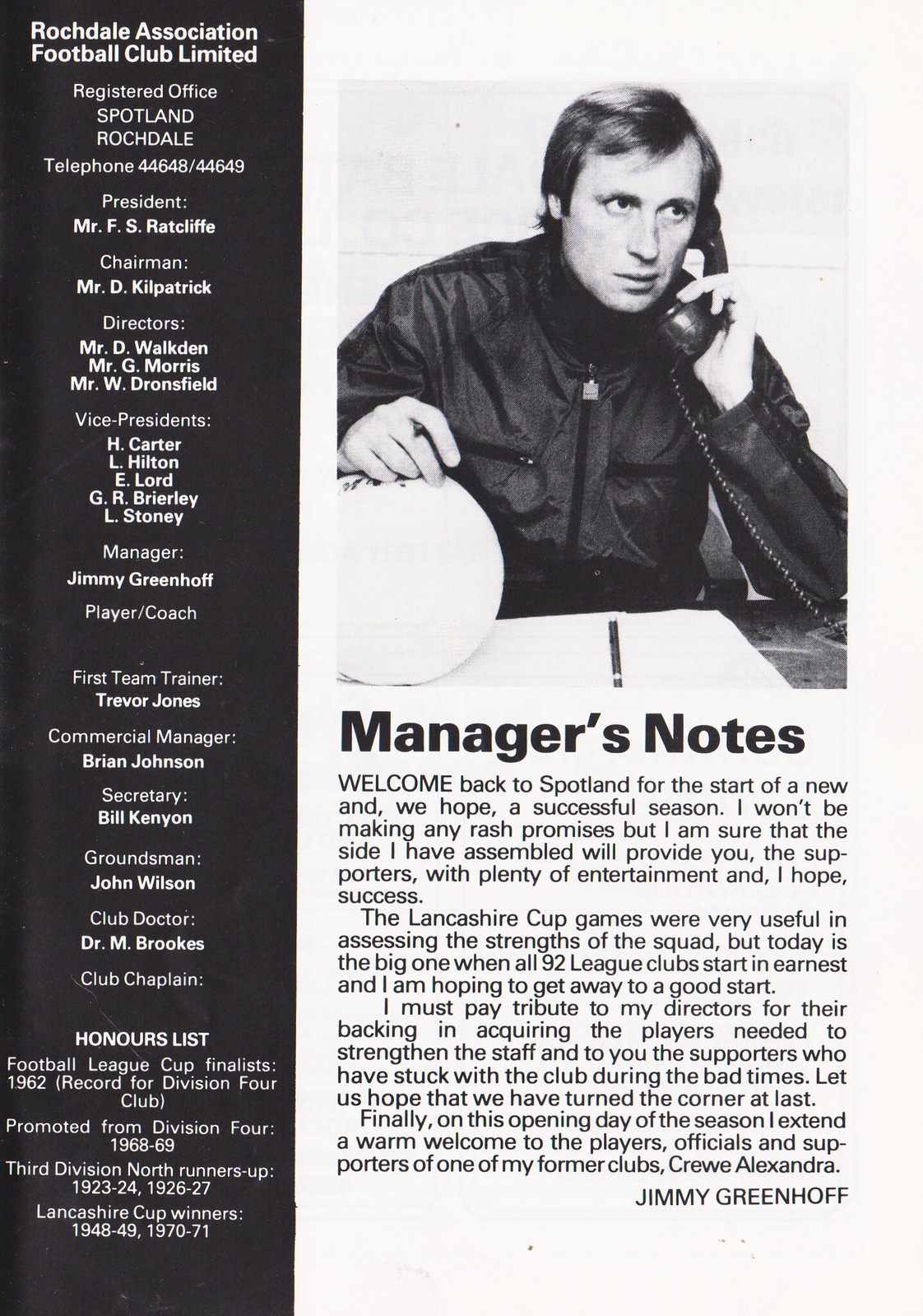The image depicts a page from a magazine, likely focusing on the Rochdale Association Football Club. Dominating the left side is a large black vertical rectangle, filled with white text detailing the club's information, including the registered office, a contact number, and a list of key personnel such as the President, Mr. F.S. Ratcliffe, and Chairman, Mr. D. Kilpatrick. Readers also find the names of other directors and various club roles such as the coach, first-team trainer, and groundsman.

On the right side against a white background, there's a large black-and-white photograph of a man, presumably the club manager, Jimmy Greenhoff. He is seated at a desk, holding a corded telephone to his ear and poised to take notes with a pen in hand. Below the photo, in bold text, it reads "Manager's Notes" followed by a welcoming message: "Welcome back to Spotland for the start of a new, and we hope, successful season." The manager addresses fans directly, expressing optimism about the season and thanking both the directors for their support in acquiring players and the fans for their steadfast loyalty. He mentions the usefulness of the Lanshire Cup games in assessing the squad's strengths and emphasizes the significance of this opening day, welcoming players, officials, and supporters of visiting clubs, specifically Crewe Alexandra. The page exudes a sense of anticipation and community spirit as the club looks forward to a promising season.